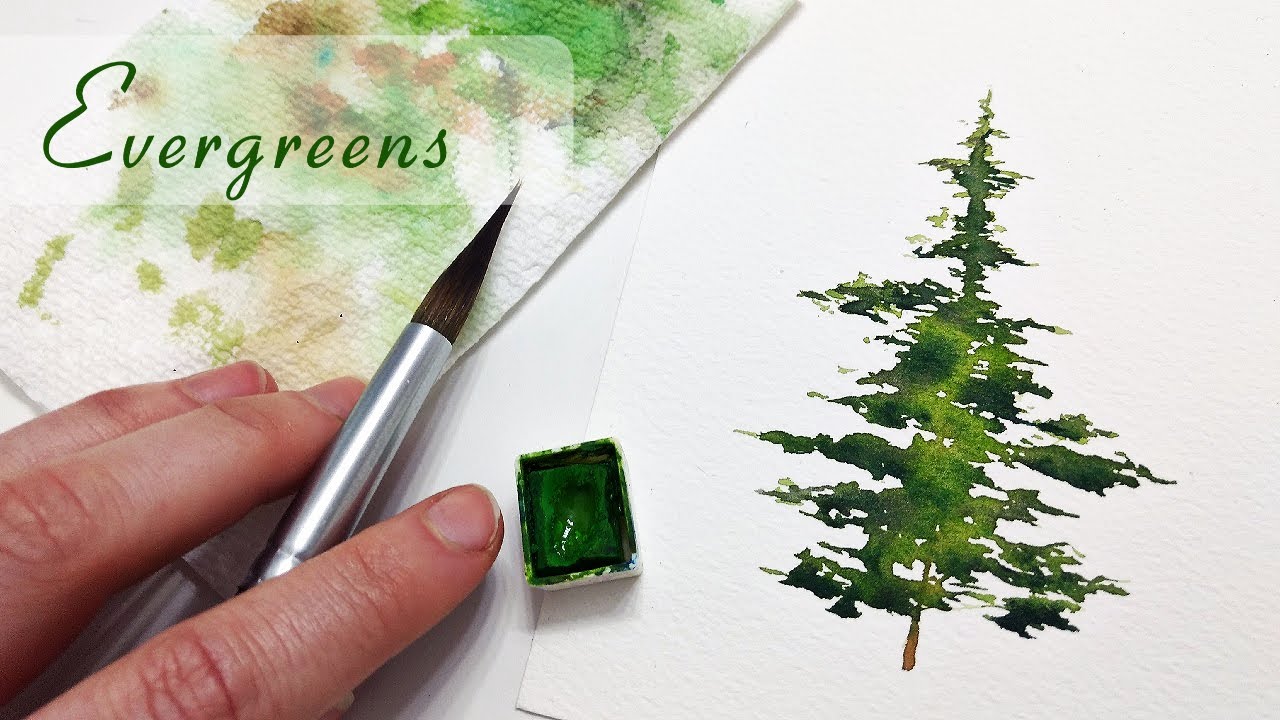The meticulously clear and well-lit photograph presents a close-up scene primarily focused on a person's left hand, appearing from the lower left corner of the horizontal rectangular frame. The individual, likely Caucasian and possibly a woman around the age of 45 to 55, is holding a shiny metal pen-like brush with a fine tip, suggesting meticulous handiwork. Extending forward from the hand, just in front of the index finger, there is a small plastic cube containing green watercolor paint. On the right side of the image, a painted evergreen tree adorns a white canvas sheet, revealing the artist's work in progress. Adding to the scene, on the top left corner lies a paper towel or blotter paper with varied green splotches—indicating recent use for adjusting shades—and some brown blotches probably used for the tree trunk. The upper left corner of the image also features the word "Evergreens" written in green letters.